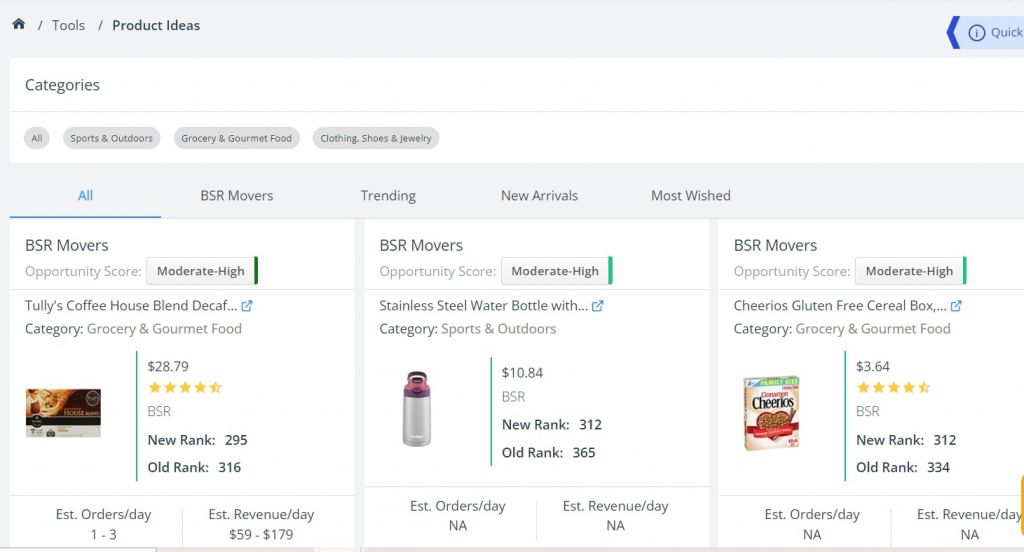This screenshot displays three products arranged horizontally in a single row, with each product occupying its own panel. The first panel showcases "Tully's Coffeehouse Blend Decaf," priced at $28.79. The second panel features a stainless steel water bottle, available for $10.84. The third panel presents a gluten-free Cheerios cereal box, priced at $3.64. At the top of the page, the word "Tools" is prominently displayed, followed by the phrase "Product Ideas." Below these headers is a section labeled "Categories" with tabs for navigating different sections such as "Sports and Outdoors," "Grocery and Gourmet Food," "Clothing, Shoes, and Jewelry." Each of these products is identified as a "BSR Mover," which may indicate a type of product ranking on this e-commerce platform. The opportunity score for these items ranges from moderate to high.